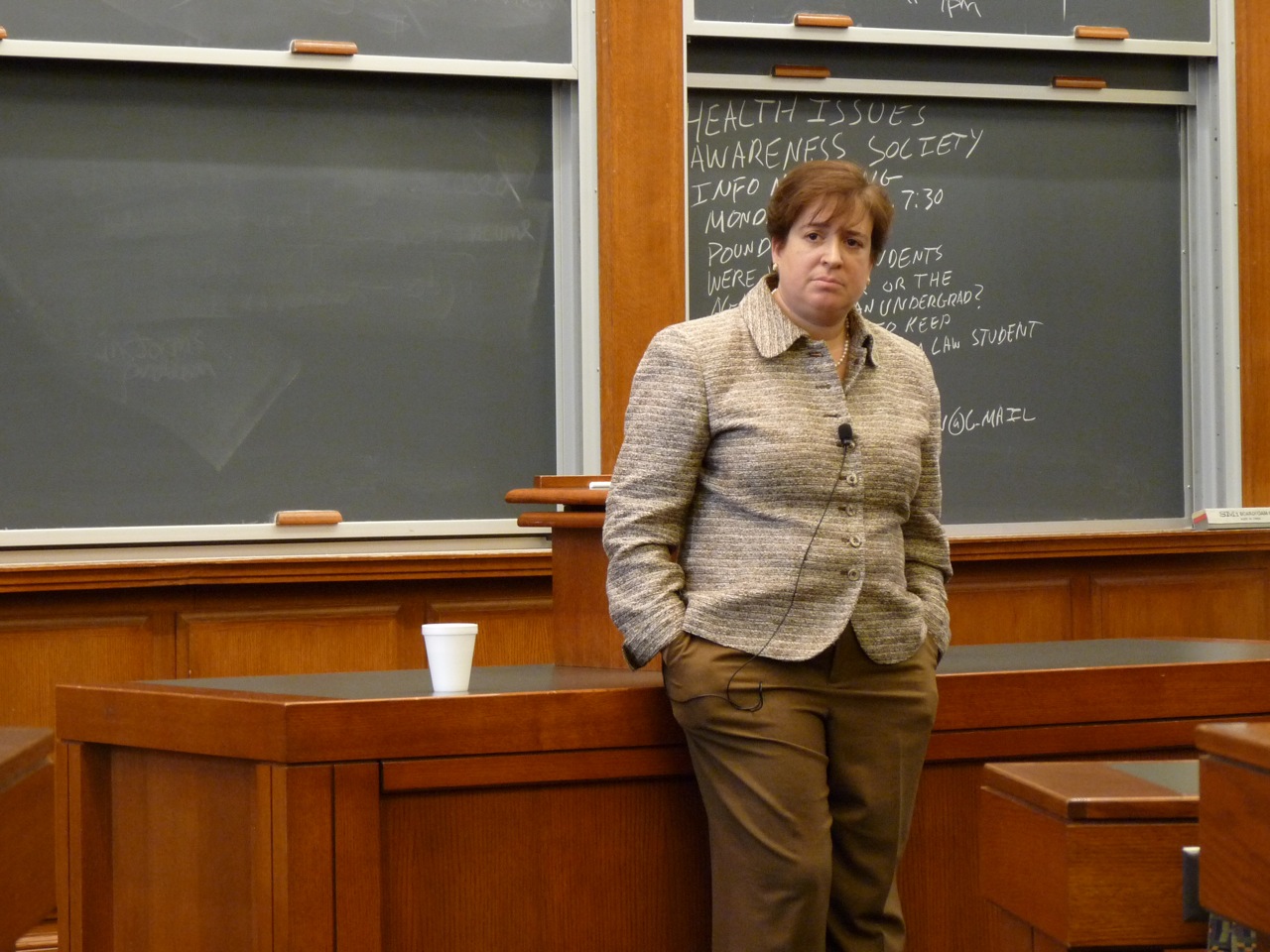In this photograph, Supreme Court Justice Elena Kagan is depicted in a classroom setting, delivering a lecture. She stands slightly to the right of the image, positioned in front of a wooden lectern. The background shows two blackboards; the one directly behind her is partially obscured by her presence and is filled with handwritten notes in white chalk, while the other remains blank. 

Justice Kagan is dressed conservatively, wearing long brown pants and a light brownish-yellow blouse, which is buttoned down. A pearl necklace adorns her neck, and she has a short haircut with bangs that frame her forehead. Attached to her blouse is a black lapel microphone, running from her pocket up to a button on her chest, hinting at her engagement in a speaking session. A white styrofoam cup is placed on the lectern's wooden base to her right. 

In this moment, she is looking attentively at someone behind the camera, perhaps a student or another participant in the room. The setting and her focused expression capture a scene of intellectual engagement and judicial insight.